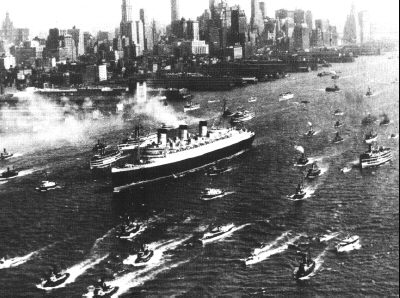This authentic black-and-white aerial photograph captures a bustling maritime scene, likely New York Harbor, from an elevated vantage point. The foreground prominently features a large body of water, filled with numerous small boats, suggesting either a river, bay, or ocean inlet. These boats appear to be centered around an imposing passenger liner with three smokestacks, reminiscent of grand ocean liners like the Titanic or the Queen Mary, though not definitively identified as either. The liner, characterized by its white top and black bottom, is releasing white smoke from its smokestacks, which drifts leftward across the image. The smaller boats seem to be either escorting or welcoming the larger ship as they all navigate towards the lower left of the frame, creating rippling wakes on the water’s surface.

In the background, the skyline of a large city is visible, with tall office buildings and old docks jutting out from the shoreline, suggesting a historical urban landscape. The photograph, likely taken from either the Brooklyn or New Jersey side, showcases a fascinating vintage perspective of maritime activity against the backdrop of an iconic cityscape, possibly that of Manhattan. The overall ambiance of the photograph evokes a sense of nostalgia, emphasizing the grandeur and historical significance of the scene captured.